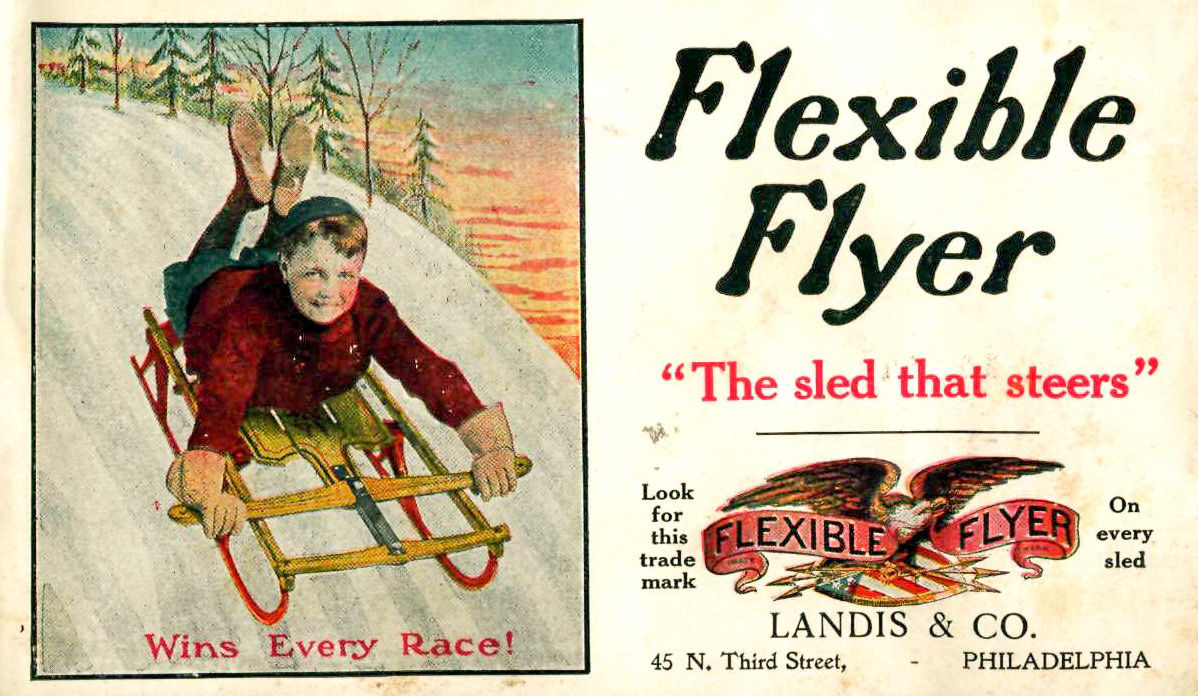This vintage poster, possibly an old advertisement, features a nostalgic cream-colored background and is divided into two main sections. On the left side, there's an illustration of a young boy sledding down a snow-covered slope with trees in the background. Below the boy, the text reads "Wins Every Race." To the right of the illustration, the heading prominently displays "Flexible Flyer" in slanted black blocky letters, followed by the tagline "The Sled That Steers" in red. Beneath this, the company's logo features an eagle clutching an American flag, and "Flexible Flyer" is written on a red banner. Flanking the logo, the text advises, "Look for this trademark," and "On Every Sled." At the bottom, the company information reads "Landis & Company, 45 North 3rd Street, Philadelphia." The majority of the text is in black, with key phrases highlighted in red.